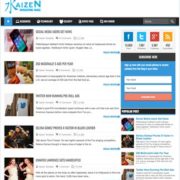The image depicts the homepage of the Kaizem (spelled K-A-I-Z-E-M) website. The Kaizem logo, located in the top-left corner, is followed by some text that is indistinguishable due to blurriness. Below the logo, five images are arranged horizontally, although the fifth image is slightly cut off. 

The first image features a person holding a black phone in their left hand, with the phone's screen displaying a predominantly blue background. To the right of this image, there is a text section consisting of a title, three smaller words or links, and a short paragraph. 

The second image appears to include a cat, with a similar text format beside it. The details of the third image are unclear. The fourth and fifth images seem to show people, each accompanied by the same text layout. Notably, all text sections adjacent to the images feature blue-colored font, except for the partially cut-off fifth image.

On the right-hand side of the page, several social media icons are displayed. Below these icons, there is a blue box containing two fields for data input and an orange submit button. Additionally, four articles, each with accompanying images, are listed on the right side of the page.